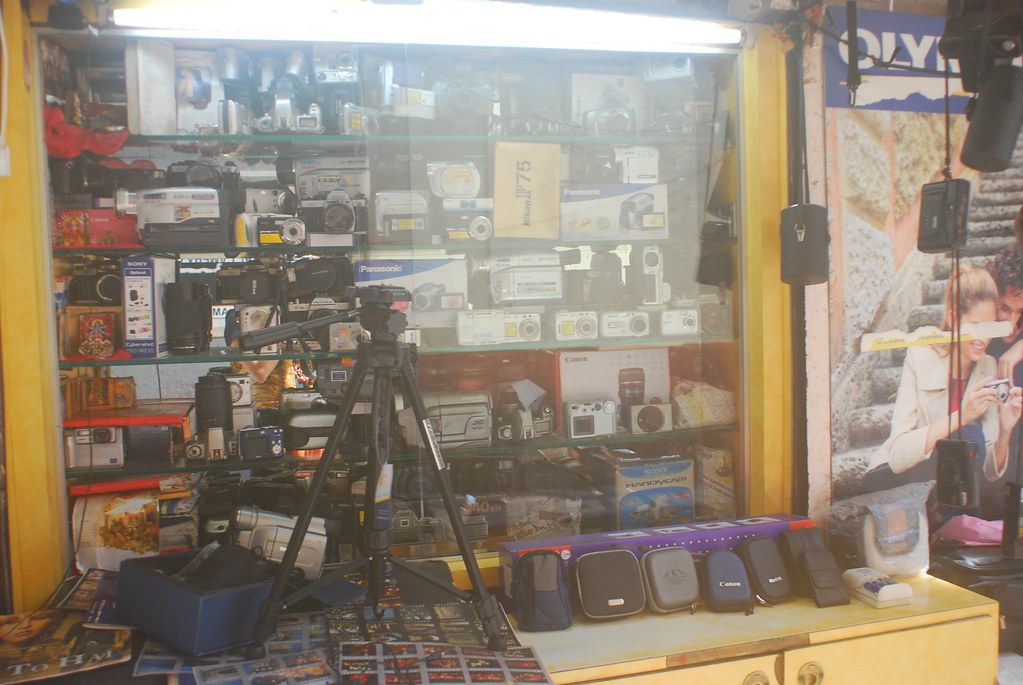The image captures an out-of-focus interior of a nostalgically dated camera shop, reminiscent of the late '90s to early 2000s. The shop features a prominent display embedded into the wall—a glass case showcasing multiple boxed and unboxed digital cameras, camcorders using micro-cassettes, various lenses, and other camera equipment. The cabinet includes six levels of glass shelves, each filled with an assortment of photography gear. The window display is framed in yellow and lit by a long fluorescent light, adding to the retro ambiance. Outside this main display case, there are additional tables set up with more camera equipment and boxes, one of which prominently displays the Canon logo. Among the scattered items, which include tripods and sheets resembling baseball cards, an easel for photographers is also visible, further emphasizing the store's focus on photographic tools and accessories.